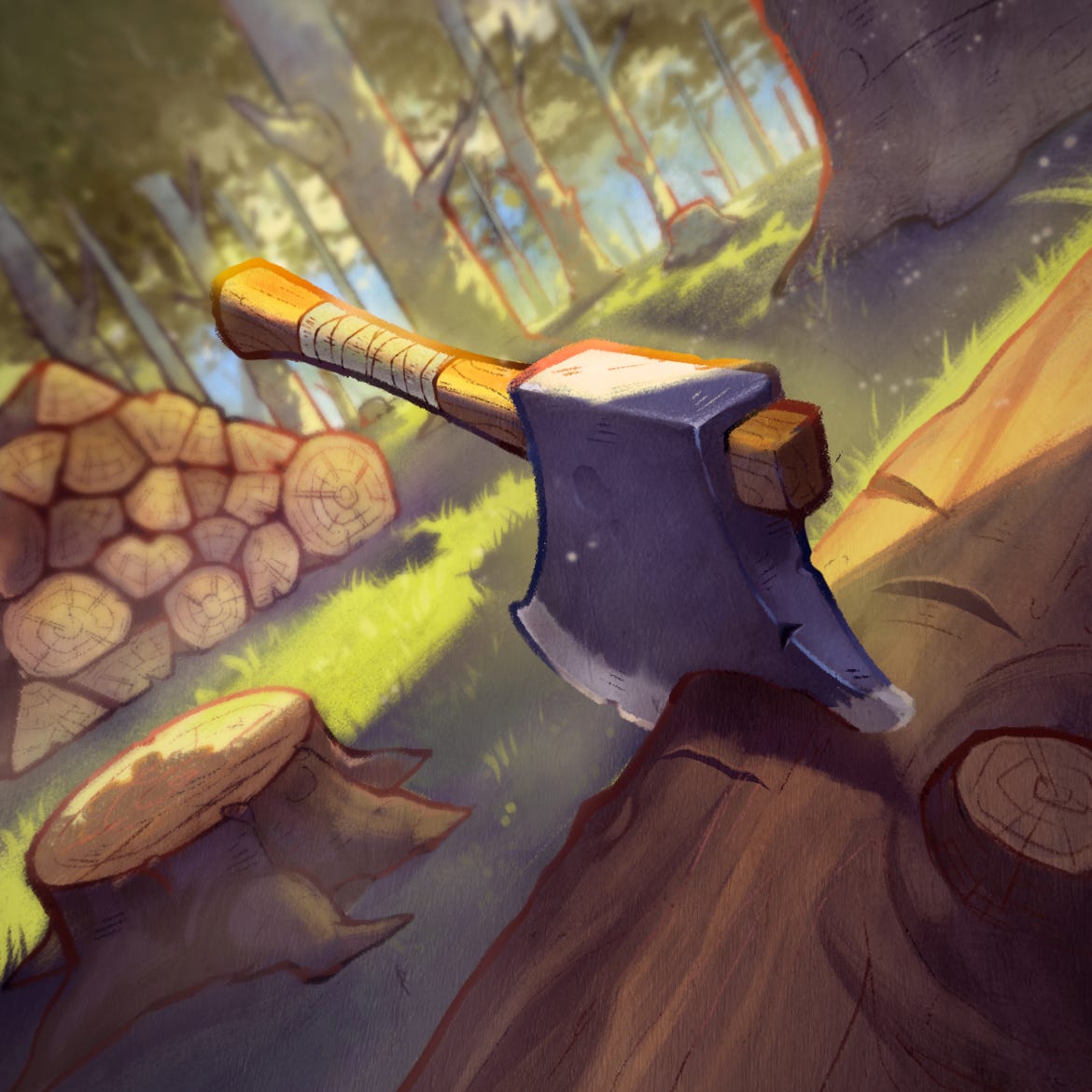The image is a cartoon-style illustration depicting a pastoral scene. In the foreground, a brown wooden log lies horizontally on a grassy field. Embedded in the log is a gray axe, with a blade that transitions from dark gray to light gray. The handle of the axe is made of wood, partially wrapped in white cloth tape for grip. 

Behind the log, a tree stump indicates where a tree was recently cut down, surrounded by a neatly stacked pile of chopped wood. The background is populated by tall, verdant trees with lush green leaves. The grass on the ground is also green, and the sunlight is prominently shining, casting a bright reflection on the grass. The overall scene exudes a sense of fresh, vibrant nature on a sunny day.